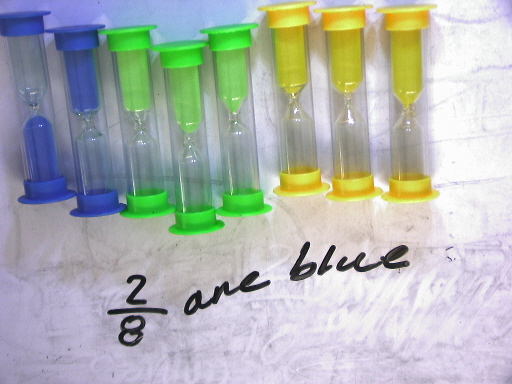This image is a top-down view of eight small plastic hourglasses, each containing sand to measure short intervals, likely in seconds. The hourglasses are color-coded: two are blue, three are neon green, and three are neon yellow. Notably, all the sand is on the top in each timer except for one blue hourglass on the far left, where the sand has settled at the bottom. Below these hourglasses, written in black Sharpie on what appears to be a dirty plastic surface or a whiteboard, there is a fraction "2/8" with the word "blue," indicating a math problem likely asking what fraction or percentage of the total is represented by the blue hourglasses. The hourglasses are unevenly lined up in a wavy pattern on the white marble-like surface they rest on.